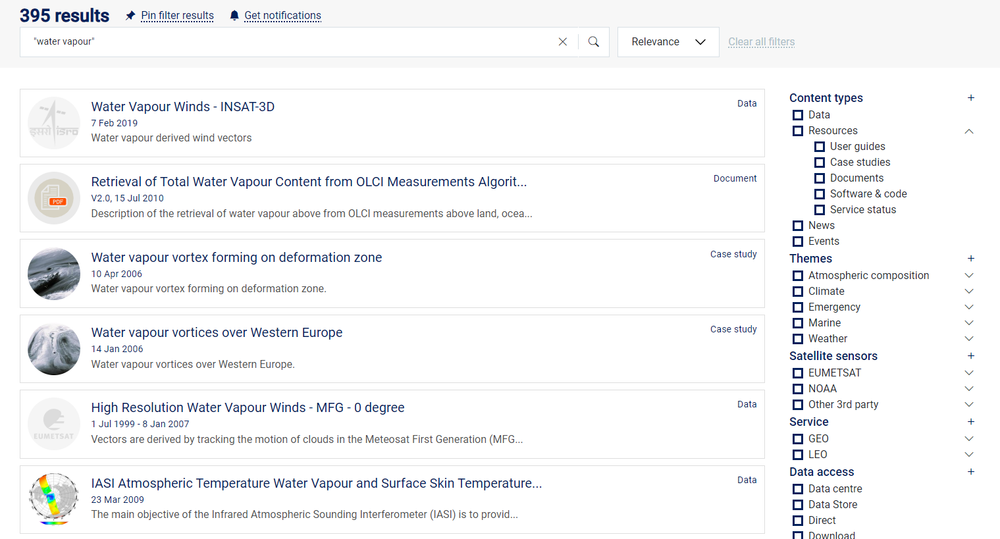This webpage from the website "395 Results" features a grayish border with black or dark blue text. At the top, there is a pin icon accompanied by the text "Pin Filter Results," and next to it, a notification icon with the text "Get Notifications." Below these icons is a search bar, within which the term "water vapor" is entered. To the right of the search bar, there is a relevance box with a drop-down arrow, followed by a "Clear All Filters" link.

On the left side of the page are several entries related to water vapor:

1. **Water Vapor Winds - INSAT-3D** - Below this title, it mentions water vapor derived wind vectors.
2. **Retrieval of Total Water Vapor Content from OLCI Measurements** - This entry is labeled as a document, focusing on an algorithm (indicated by ellipses).
3. **Water Vapor Vortex Forming on Deformation Zone (10 April 2006)** - Marked as a case study, discussing the formation of water vapor vortices on that date.
4. **Water Vapor Vortices Over Western Europe (14 January 2006)** - Another case study examining water vapor vortices over Western Europe.
5. **High-Resolution Water Vapor Winds - MFG 0 Degree (1 July 1999 - 8 January 2007)** - Vectors derived by tracking the motion of clouds in the METEOSAT First Generation (MFG), categorized as data.
6. **IASI Atmospheric Temperature, Water Vapor, and Surface Skin Temperature (23 March 2009)** - Described as data, with a focus on the infrared atmospheric sounding interferometer (IASI) and its main objective (again, indicated by ellipses).

On the right side of the page, various content types are available, each with a drop-down arrow:
- Data Resources
- User Guides
- Case Studies
- Documents
- Software and Codes
- Service Status

Additional categories such as News, Events, and Themes include:
- Atmospheric Composition
- Climate Emergency
- Marine Weather
- Satellite Sensors (EUMETSAT, NOAA, other third party)
- Service (GEO, LEO)
- Data Access (Data Center, Data Store, Direct, and Download)